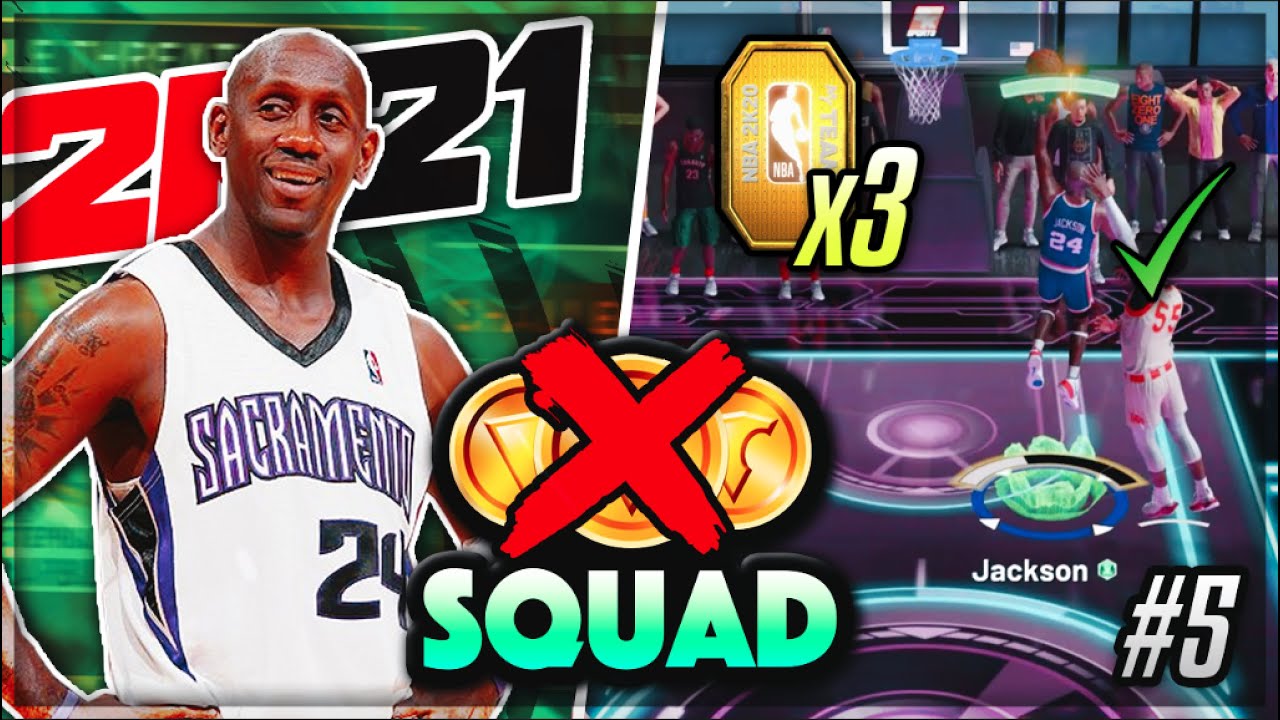The image appears to be a screenshot from an NBA video game, possibly showing a player from the Sacramento Kings. The focal point is a close-up of a player wearing a jersey with the number 24. He has visible tattoos on his arms, his hands on his hips, and a smile on his face, suggesting he is pleased or confident. His skin glistens with sweat, indicating active gameplay.

In the background, there is a graphic featuring the year "2021," with "20" in red and "21" in black, both numbers outlined in white. The overall color scheme behind the player is predominantly green, possibly to match the trim of the player's jersey around the neck.

Centrally, there's a prominent red "X" with the word "SQUAD" in all capital letters below it, the letters having a greenish hue. To the right, there is text that reads "Jackson number 5," and in the upper corner, there's an interface element showing "times 3 for the tickets," along with a green check mark, indicative of a reward or achievement within the game.